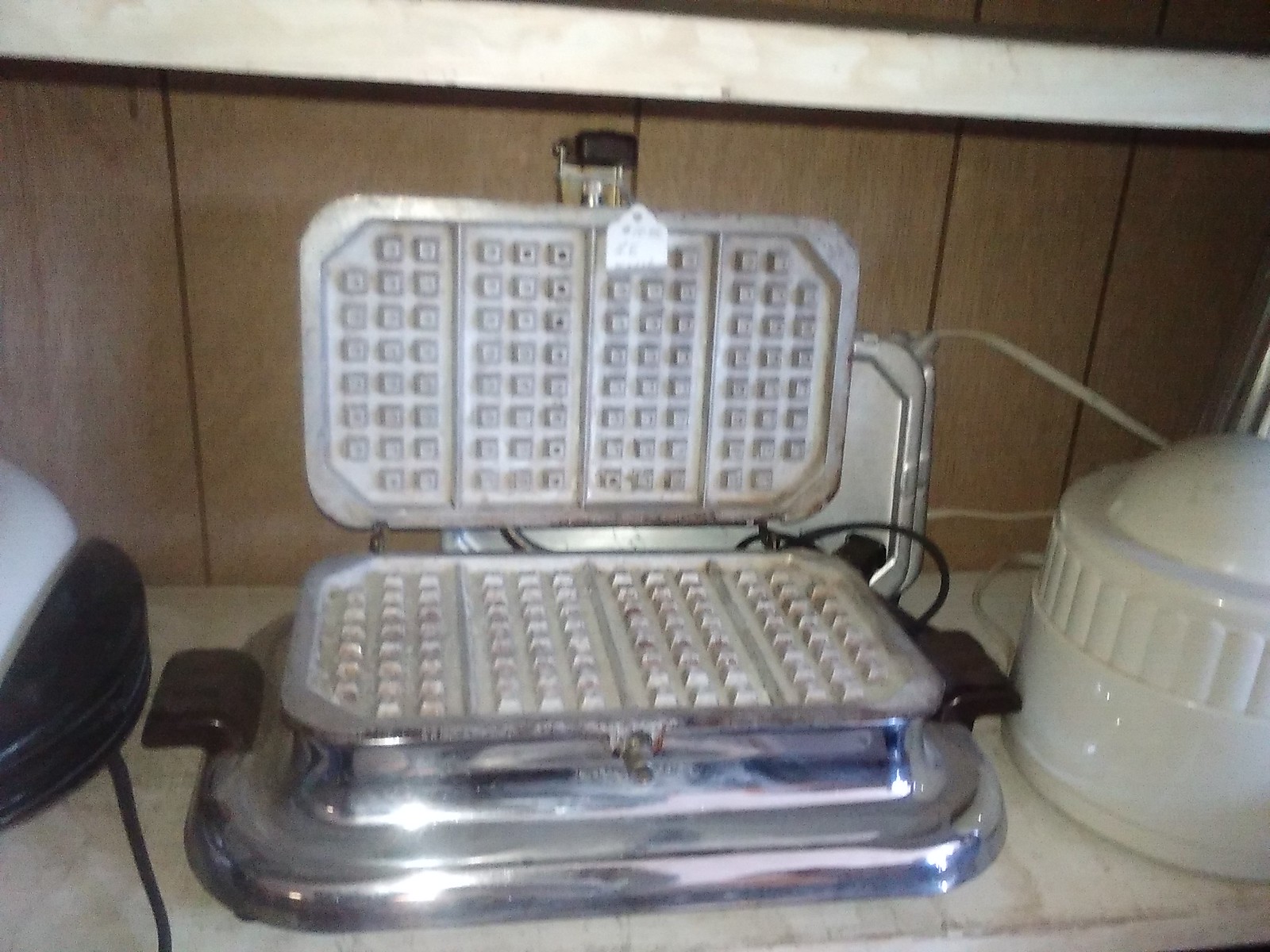The photograph is a colour close-up shot in a kitchen, focusing primarily on an open rectangular metal waffle maker with a shiny, reflective chrome exterior. The waffle maker has a grid pattern of raised square pieces on both the top and bottom plates, designed to form waffles. It features black handles on its base and appears to be placed on a white shelf with an electrical cord extending from it. The shelf is affixed to a wall lined with vertically running wooden panels, displaying visible gaps between them. To the left of the waffle maker, only a portion of another kitchen device is visible, identifiable by a black handle and a white section, likely a lid of some roasting appliance. On the right side of the waffle maker sits a white ceramic container with a detachable lid. Above this shelf, the lip of another shelf is visible, creating a subtle angle down to the waffle maker below, though its contents are not visible in the frame.